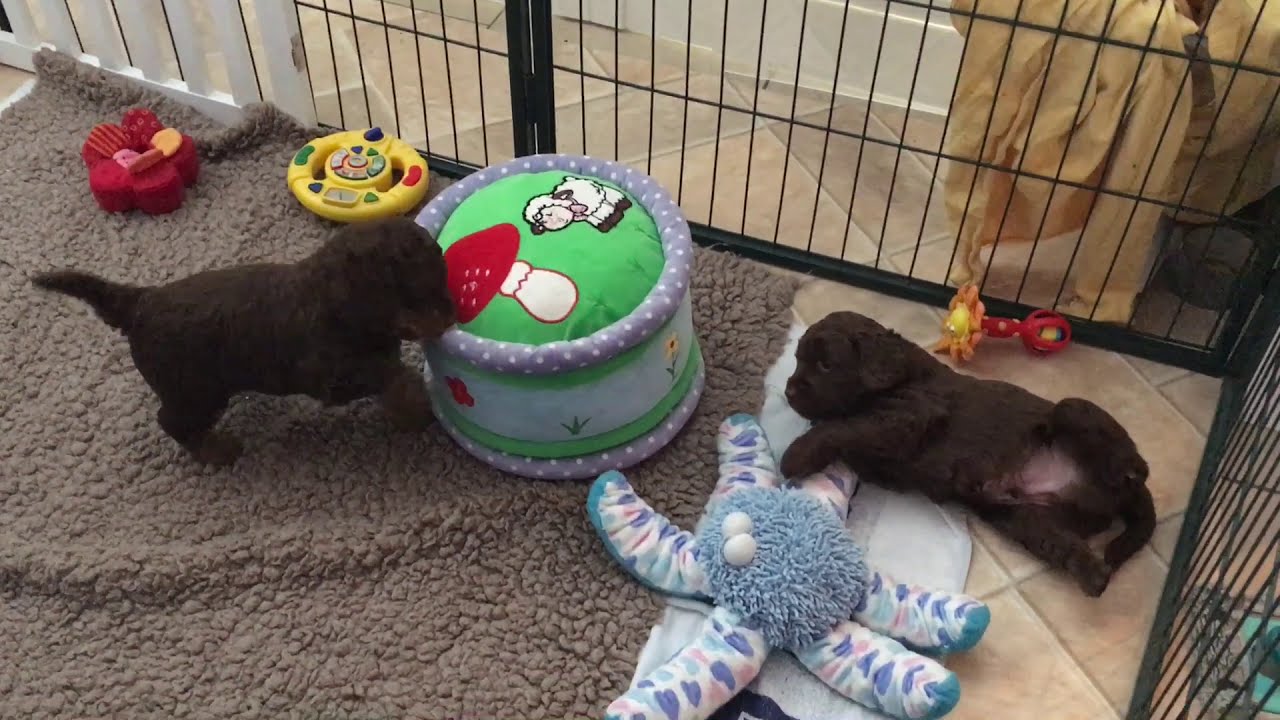The photograph depicts an indoor scene featuring two small, completely brown puppies within a black metal gate enclosure on a beige tile floor. The enclosure includes a light brown furry carpet. One puppy is lying on its back, exposing its pink belly, while the other is standing, sniffing a small round cushion decorated with a green top and a red mushroom cap surrounded by a lavender edge with dots. The enclosure contains various toys, notably a blue octopus-like toy and several others that resemble children’s toys. Additional toys include a yellow item with buttons and a red flower-shaped toy. The setting, which might be a home or a veterinarian's office, reveals a baseboard behind the enclosure and fabric hanging to the right. The detailed realism of the photograph captures both the playful energy and the cozy environment created for the puppies.